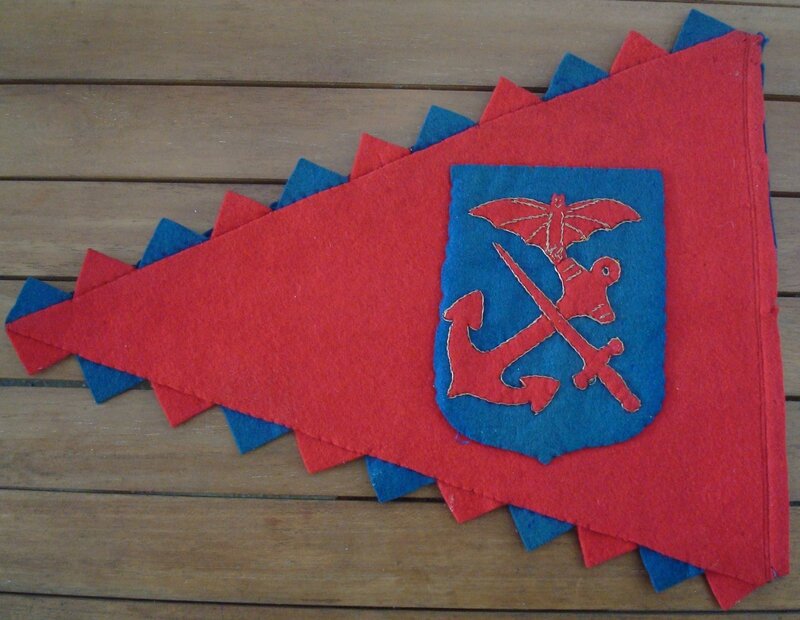This is a detailed color photograph in landscape orientation, showcasing a handcrafted felt pennant laid against a light to medium brown wooden deck composed of horizontal planks. The pennant, made from red fabric, is triangular in shape with its point directed to the left side of the image. Along the top and bottom edges of the pennant are alternating red and blue triangles that add decorative flair. At the center of the pennant is a blue shield, embroidered or sewn onto the fabric. The shield features a red bat with outstretched wings at the top, and below it, an anchor and sword crossed at the bottom, both in red. The crafted felt pennant reflects detailed artistry and the photographic style captures this representationally.